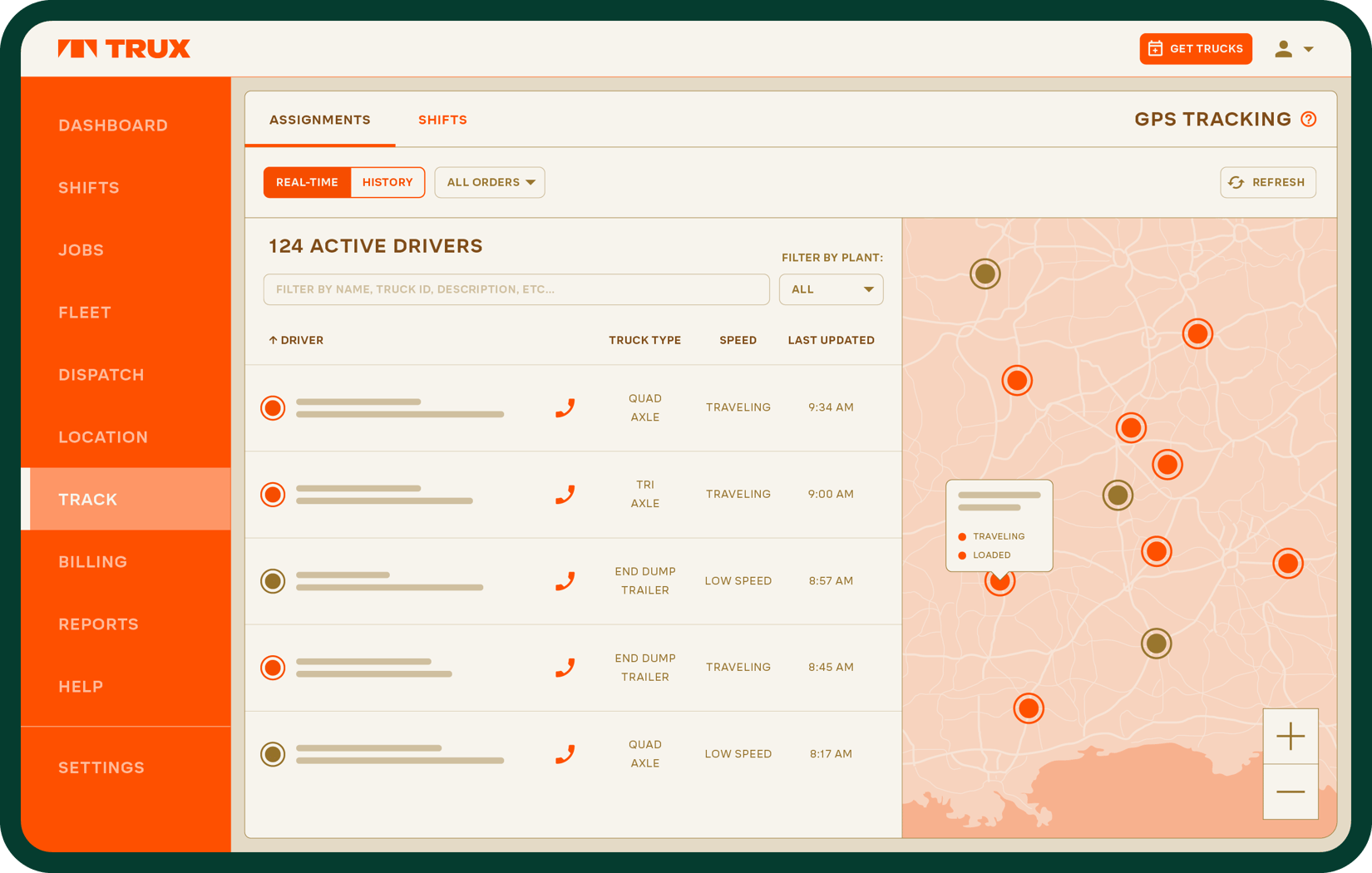This screen capture displays a vividly designed website centered around fleet management. The website, adorned with a predominantly orange and tan color scheme complemented by brown fonts, features a tan navigation bar at the top. This bar prominently displays the site name "Orange Trucks." Adjacent to this is an orange and white button labeled "Get Trucks," accompanied by a calendar icon and a brown pull-down icon representing a user profile.

To the left, there's an orange sidebar hosting white submenu options such as "Dashboard," "Shifts," "Jobs," "Fleet," "Dispatch," "Location," and "Track." The current section, "Track," is highlighted with white text on a light orange background. Further options include "Billing," "Reports," "Help," and "Settings."

In the central panel, headers in brown and orange fonts indicate sections like "Assignments" and "Shifts." Below these headers, an orange bar delineates real-time statuses, displaying "Real-Time," "History," and "All Orders." Beneath this, there's text indicating "124 Active Drivers" in brown, alongside a search box for filtering by name, truck, or description. A dropdown filter labeled "Filter by Plant" is set to "All."

The main content area lists driver names, which are blurred out for privacy. Each driver entry features an orange phone icon and different truck types, including Quad Axle, TP Axle, End Dump Trailer, another End Dump Trailer, and a Lot Axle. Status indicators show varying speeds like "Traveling" and "Low Speed," with last update timestamps ranging from 8:40 AM to 9:38 AM.

The bottom portion of the screen displays an orange map dotted with orange and brown circles, indicating various locations. A plus and minus sign on the map suggests zoom control functionality.